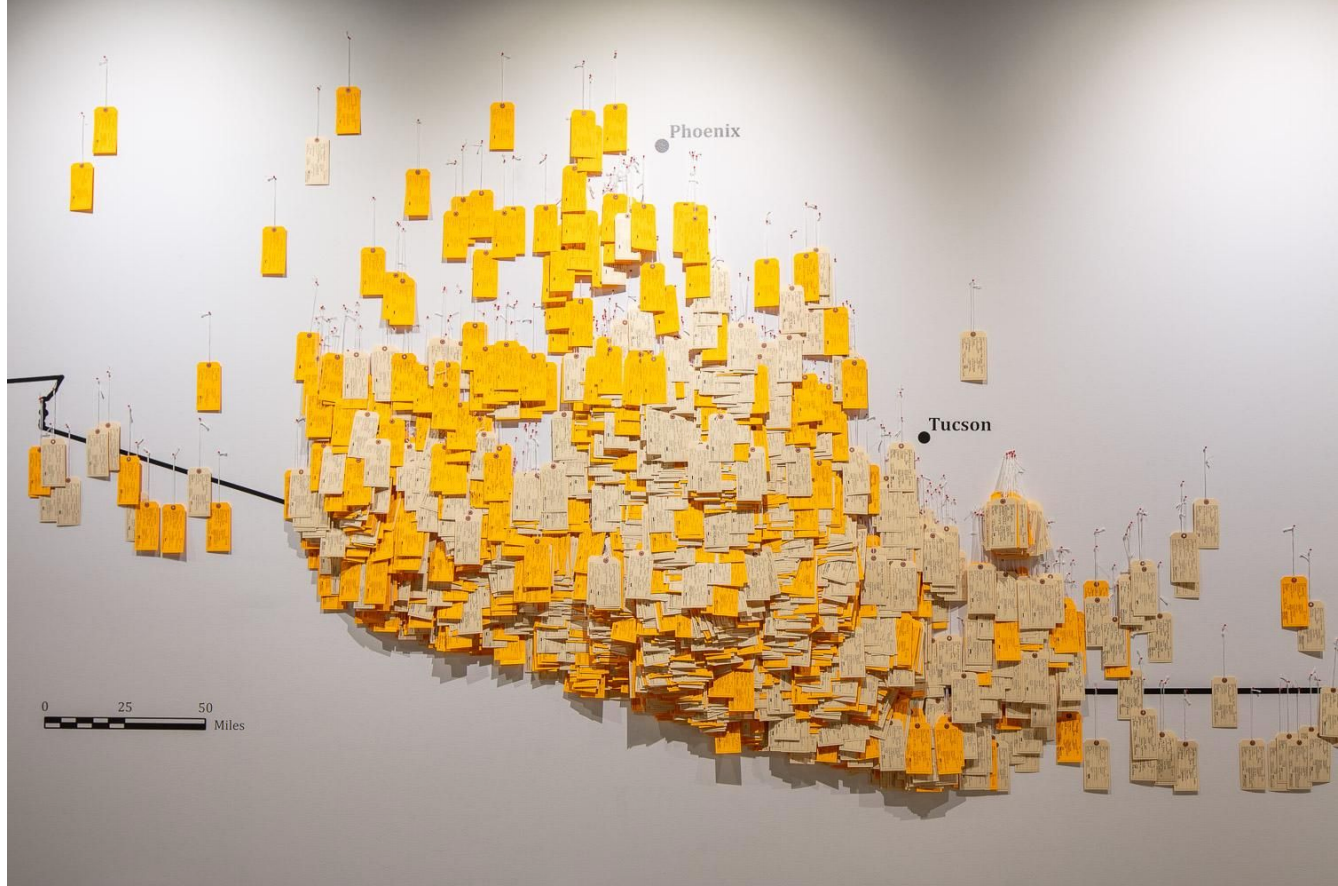The image depicts a detailed installation on a white wall, featuring a bordered map of Arizona with notable towns Phoenix and Tucson clearly marked with dots. A serpentine line, representing either a border or a route, meanders across the map, highlighted by a legend indicating distances of 0, 25, and 50 miles. Suspended from this line are hundreds of small tags resembling toe tags or travel luggage tags, in varying shades of yellow, orange, and beige. These tags, each with an eyelet and string, are densely clustered along the southern part of the map near the Mexican border, below Tucson, with a notable concentration stretching towards Phoenix. The tags, although their inscriptions are not legible from the image, create a textured and intricate visual, suggesting a significant representation of data, possibly related to migration or travel patterns. The entire installation conveys a powerful visual narrative, emphasized by focused lighting that casts soft shadows and highlights the three-dimensional aspect of the tags against the wall.